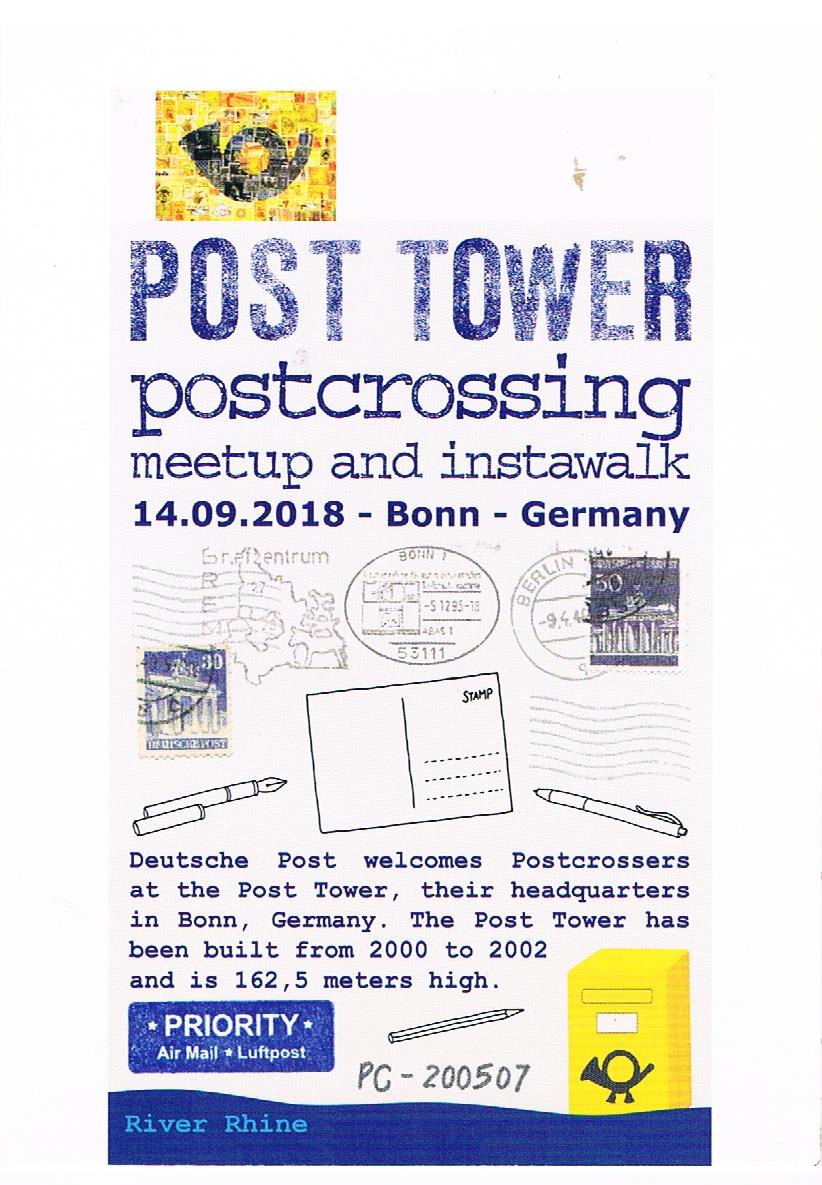The advertisement displayed on a smartphone is vertically oriented and prominently features a square box with a black postal horn and a circular round horn. Blue text reads "Post Tower Post Crossing Meetup InstaWalk 14.09.2018 / Bonn, Germany." The composition includes distinct German postal stamps depicting Berlin, along with illustrated pens and a postcard in the center. Below, blue text states, "Deutsche Post welcomes post crossers at the Post Tower, their headquarters in Bonn, Germany." The Post Tower, constructed between 2000 and 2002, stands at 162.5 meters high. Near the bottom of the image, a blue stamp mark labeled "Priority Airmail Luftpost" can be seen alongside an illustration of a pen, the code "PC-200507," and a yellow post box featuring a black horn. A blue wave inscribed "River Rhine" flows across the bottom of the image.